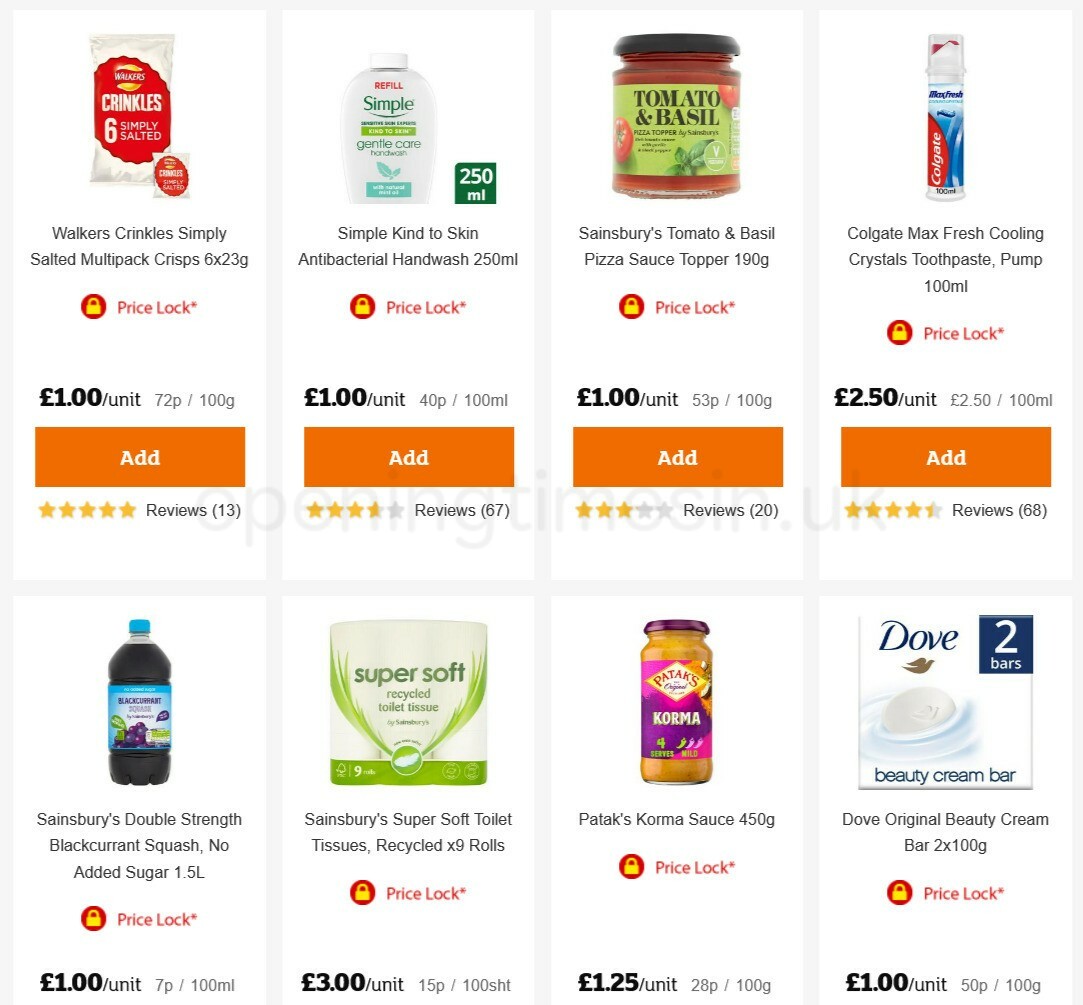This image captures a screen displaying an online shopping interface with a grid layout for product listings. The interface is split into two rows with four items per row, each following a consistent format. 

At the top, the first row includes items such as a bag of Crinkles Salted Crisps, a bottle of Antibacterial Hand Wash, a jar of Tomato Basil Sauce, and Colgate Max Fresh Cooling Crystals toothpaste. Each product entry includes a thumbnail image of the item, a brief description, and a "Price Lock" icon, indicating a fixed price, which all items display. 

Underneath each item, additional details are provided, including the unit price and quantity, such as weight in grams. An orange "Add" button is present for each product, with "Add" written in white text, suggesting the option to add these items to a virtual shopping cart.

The second row appears to follow the same format, with products like Black Currant Squash, identifiable as a liquid beverage. Each item listing continues to display the same elements as the first row: product image, description, price lock emblem, unit price, and the "Add" button.

Customer reviews and ratings are partially visible; each product has a five-star rating system where some items have only three stars lit up, while others have a complete five-star rating. However, the lower section of the screen, which includes the detailed customer reviews and possibly additional functionality related to the stars and "Add" button, is cropped out and not visible in the image. 

Overall, the screen showcases a neatly organized selection of products available for online purchase, emphasizing ease of shopping with clear item descriptions, pricing details, and customer feedback indicators.